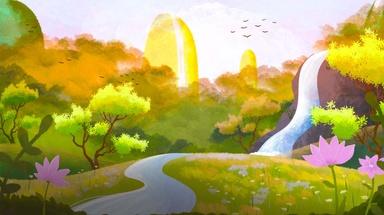This vibrant digital illustration depicts a lively nature scene with a cartoony, animated style. Dominating the background is a radiant sun, casting a warm glow over the composition. Birds swoop gracefully through the light blue sky, dotted with soft, wispy clouds. Prominent in the scene is a meandering river that originates from the upper right and winds its way to the lower left, transitioning seamlessly into a waterfall cascading towards the right.

The landscape is rich with color, almost exaggeratedly so, featuring chartreuse greens and vivid purples. The verdant fields are interspersed with various trees, showcasing both lighter and darker shades of green, highlighted with bright yellow accents. Pink flowers punctuate the corners, one on each side, adding a burst of vibrant color.

To the left side, there is a notable circular green object, while towards the far end, a tall, yellow oblong shape stands out with a smaller similar object beside it, contributing to the forest's whimsical charm. This scene captures the essence of a lush, animated countryside, brimming with exaggerated hues and a playful aesthetic.